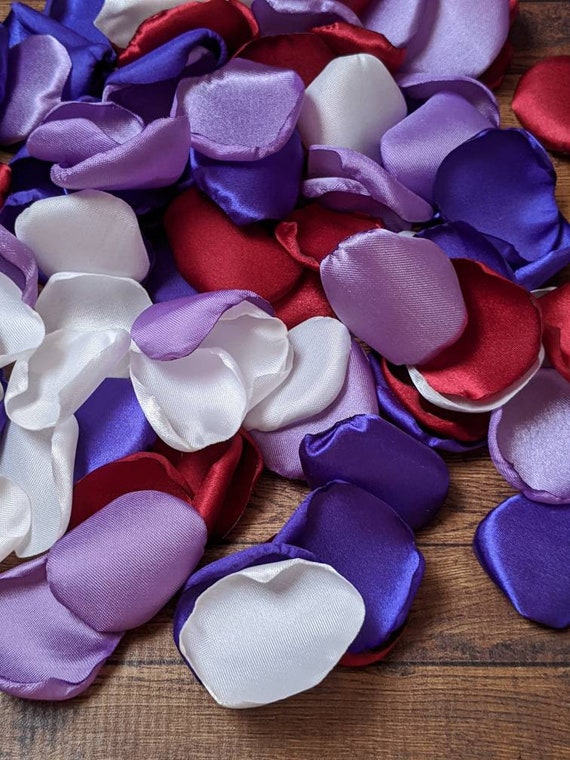This image depicts a wooden surface, likely a medium brown wood floor with dark lines delineating the planks. Scattered across this floor is a collection of fabric pieces, crafted to resemble the delicate form of rose petals. The petals, made from various shiny fabrics, are mixed in an array of colors—white, dark purple, light purple (lavender), and red. Most of these fabric petals are heaped towards the top left of the image, with a few scattered across the foreground where the surface is more visible. There appears to be around 50 to 100 petals in total, creating a vivid, colorful display that starkly contrasts against the wooden backdrop. The scene evokes the appearance of freshly fallen rose petals, albeit crafted from a luxurious, silky material.